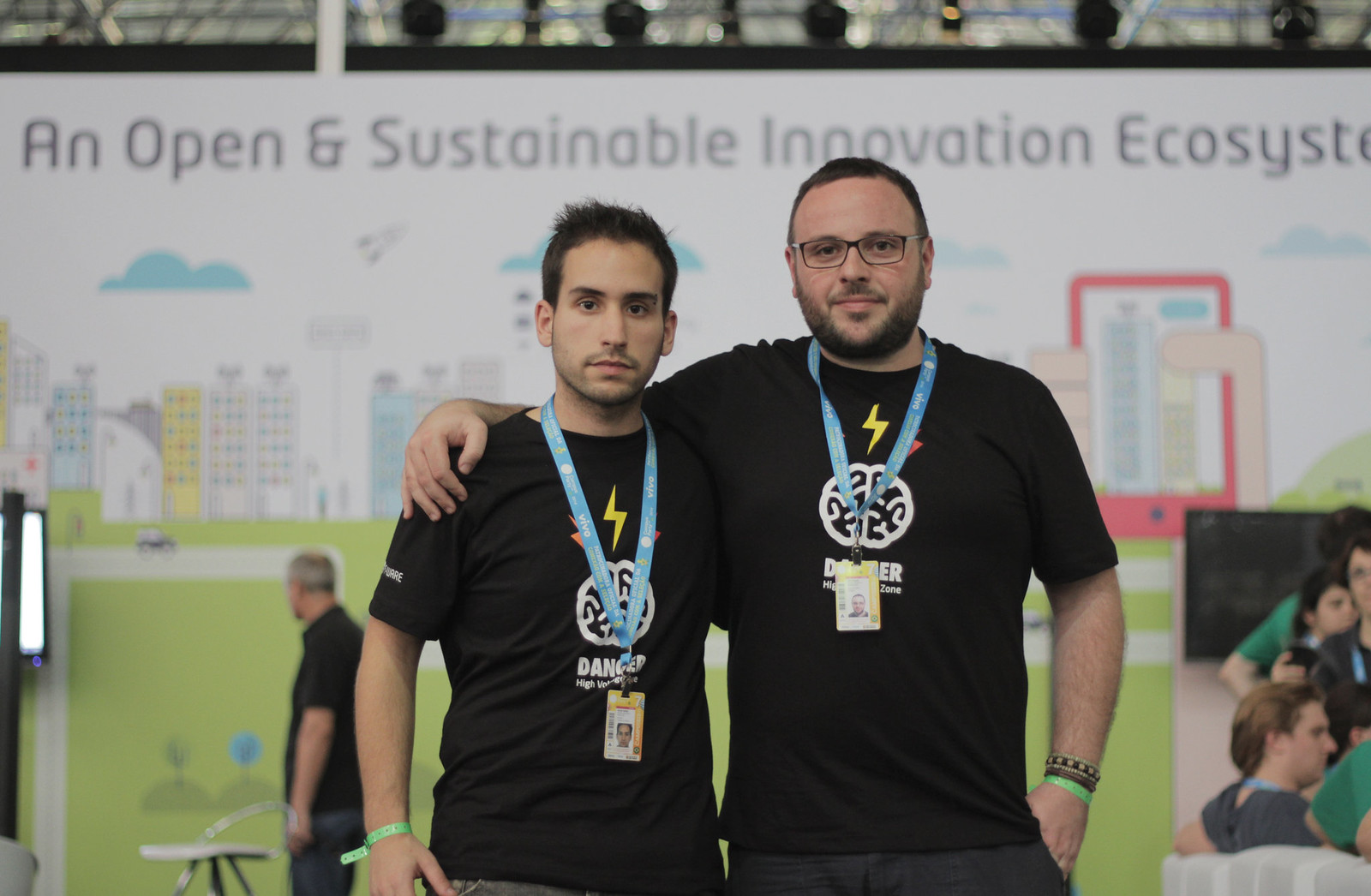In this horizontally aligned rectangular photo, two young men, likely in their 20s, stand closely together in the foreground, appearing to attend an event related to engineering or urban design. Both men wear identical black t-shirts featuring a white emblem that resembles a brain, topped with yellow, red, or orange lightning bolts, and the word "DANGER" printed in white underneath. They each have blue lanyards around their necks with ID badges attached. 

The man on the left is shorter with short dark hair, a thin mustache and beard, and a green bracelet on his right wrist. The taller man on the right has short brown hair, a thicker beard and mustache, glasses, and a green bracelet on his left wrist. His right arm rests around the shoulders of the man on the left, reflecting their camaraderie.

In the blurred background stands a wall displaying the words "An Open and Sustainable Innovation Ecosystem," accompanied by outlines of clouds, buildings, roads, and a person holding a cell phone. Additionally, to the left, there is a blurry image of a man with gray short hair wearing a black t-shirt, gazing at the mural. This meticulously detailed scene encapsulates the atmosphere of innovative collaboration and urban design.